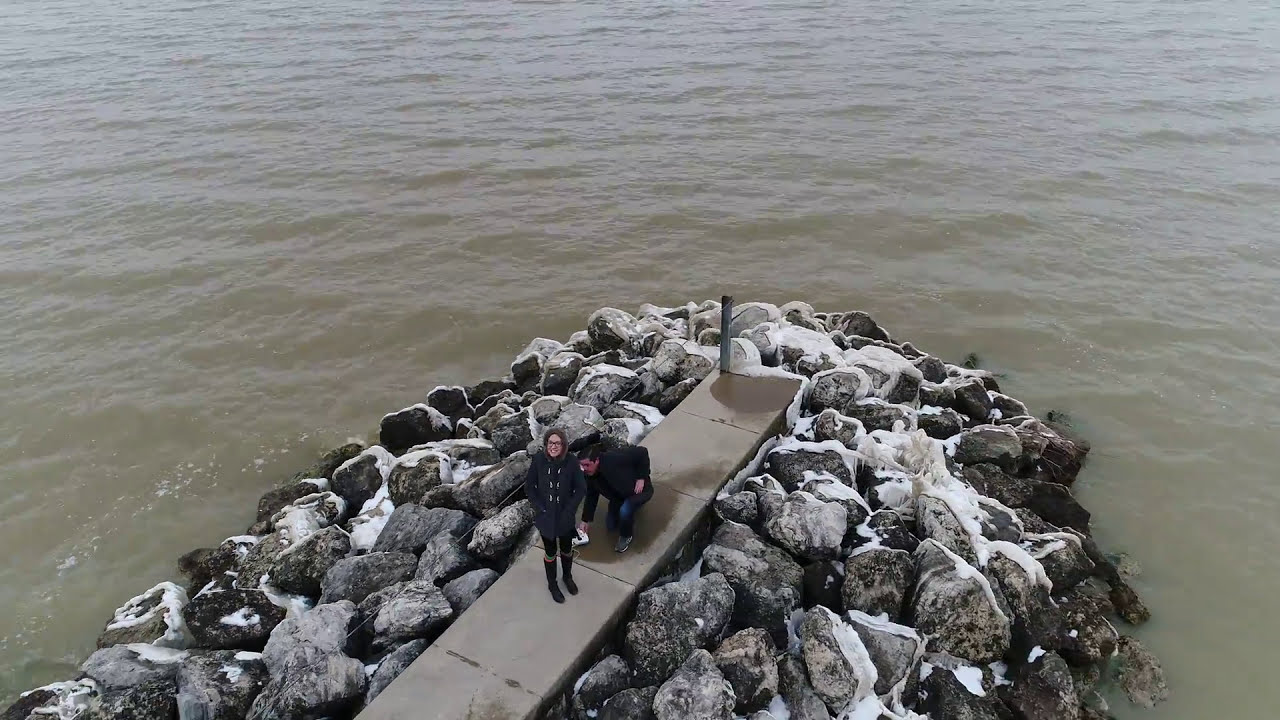A high-angle aerial shot, likely from a drone, captures a rocky outcropping or pier extending into the murky, brown waters, possibly of a Great Lake. The man-made structure consists of large rocks with patches of snow and ice, creating a rugged backdrop. Down the center runs a narrow, concrete sidewalk, bordered partially by a wire guide. Situated in the center left of the image are two individuals. The young woman, clad in a dark blue coat with her hood up and boots, stands with her hands in her pockets, looking up at the camera. Her male companion, slightly behind her, is in a black coat, jeans, and sneakers, kneeling on one knee with one hand touching the snowy ground and the other resting on his leg. The scene suggests a stormy atmosphere, with choppy waters adding to the dramatic, cold environment.